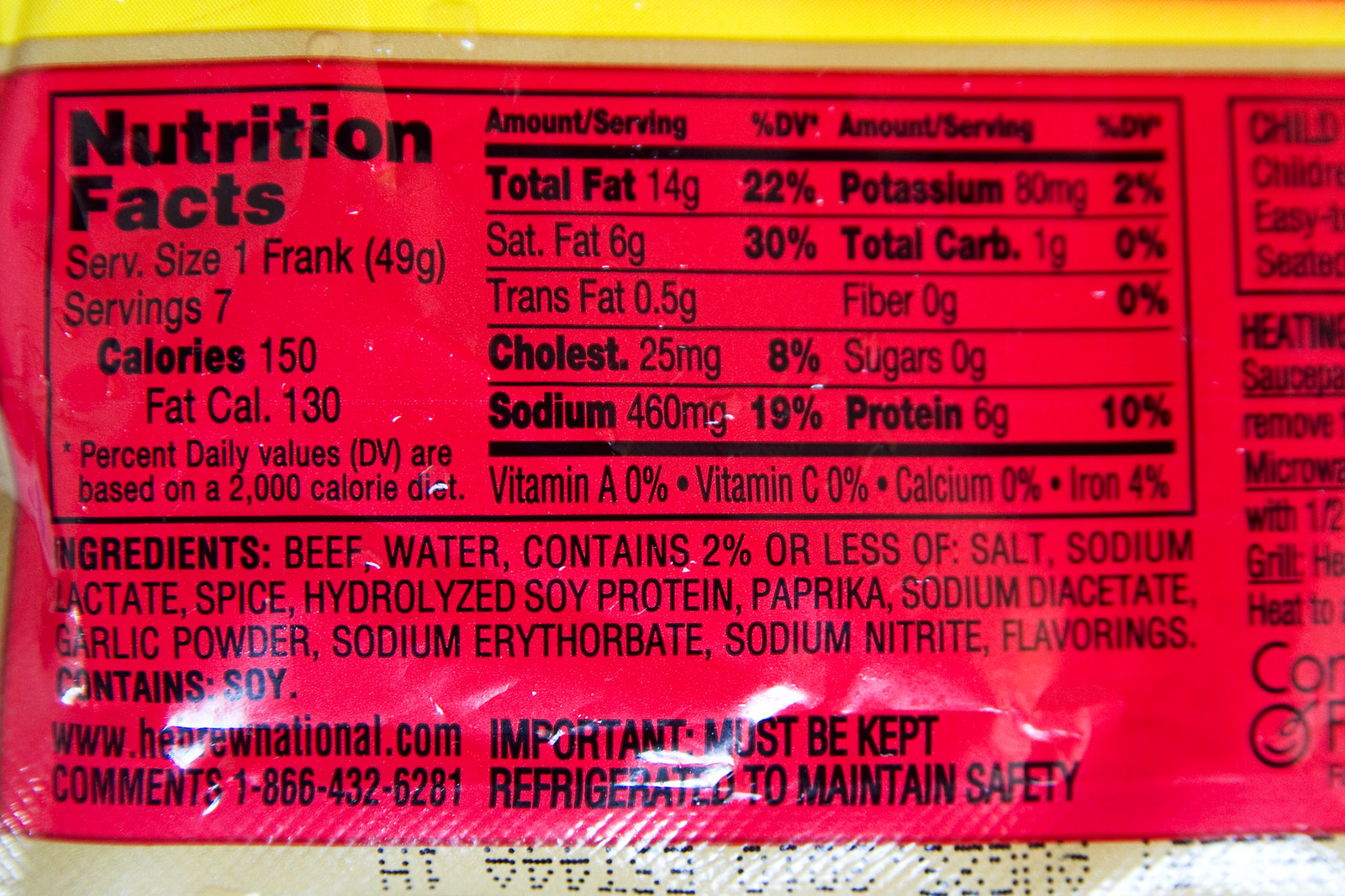The image is a close-up photograph of the nutritional label on a plastic food package, specifically a package of hot dogs. The label is set against a reddish-pink rectangular panel featuring black text. At the top of the image is a yellow line fading into orange, with a tan line beneath it, and another tan line at the bottom of the label. The label shows some folding and creasing with reflections of light making certain areas harder to read. The nutritional facts section details a serving size of one frank (49 grams), with seven servings per container. It lists 150 calories per serving, with 130 calories from fat. Nutritional information includes 14 grams of total fat (22% DV), 6 grams of saturated fat (30% DV), 0.5 grams of trans fat, 25 milligrams of cholesterol, 460 milligrams of sodium (19% DV), 80 milligrams of potassium (2% DV), 1 gram of total carbohydrates (0% DV), 0 grams of dietary fiber, 0 grams of sugar, 6 grams of protein (10% DV), 0% Vitamin A, 0% Vitamin C, 0% calcium, and 4% iron. 

The ingredients list includes beef, water, less than 2% of salt, sodium lactate, spice, hydrolyzed soy protein, paprika, sodium diacetate, garlic powder, sodium erythorbate, sodium nitrate, and flavorings. It emphasizes in bold: "Contains soy." The package also provides a web address (www.hebrewnational.com) and a contact number (1-866-432-6281), and it highlights the importance of refrigeration with the bold warning, "Must be kept refrigerated to maintain safety." Additionally, some child safety and heating instructions are partially visible. The label indicates the product is under the brand Hebrew National.